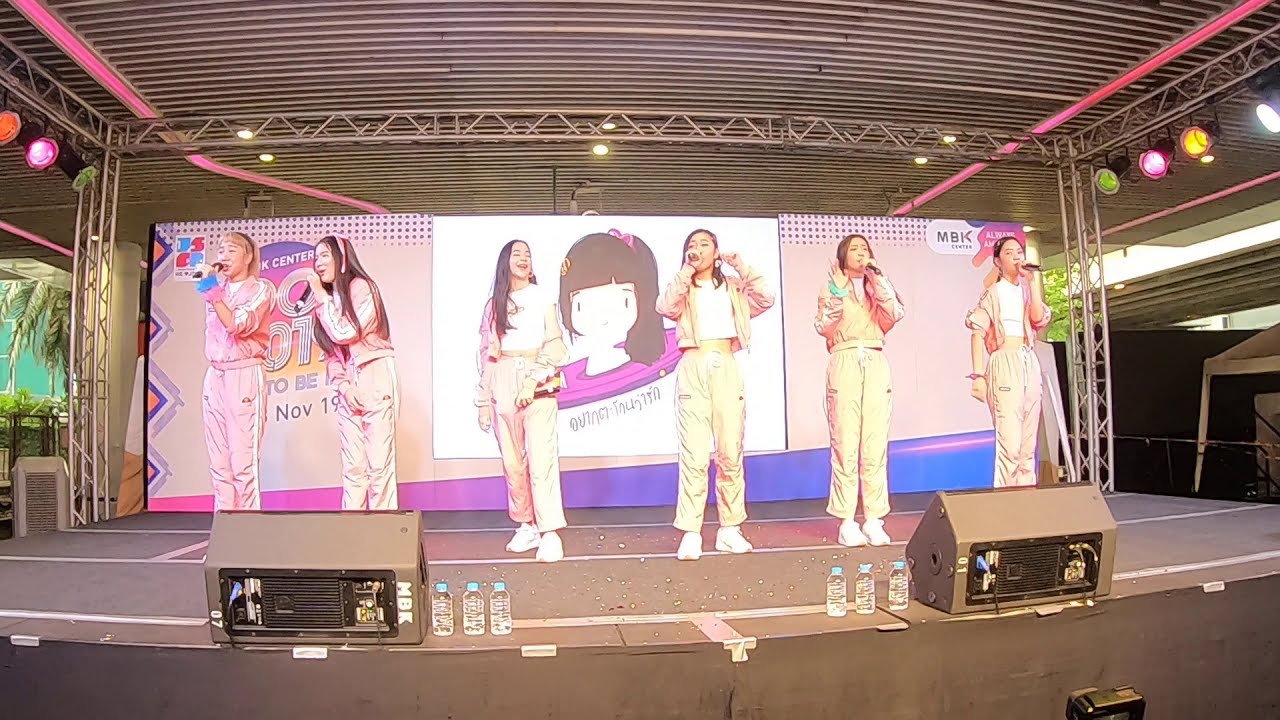Six young Asian girls, dressed in coordinated light pink tracksuit outfits, stand on a black stage adorned with white lines. They each hold a microphone, with most singing into theirs, performing under colorful spotlights of green, pink, and yellow. The backdrop features a large video screen prominently displaying an anime drawing of a girl with brown hair tied into a ponytail on the right side of her head, set against a predominantly pink background with hints of purple. These girls are centered on the stage, flanked by two large PA speakers, beside which rest three clear water bottles on each side. Above them, metal slats and lighting fixtures form a canopy, casting a vibrant illumination on the scene. In front of the singing group are two brown boxes, adding to the structured setup of the space. The left side of the backdrop includes signage about an event on November 19th. One girl stands out with her blonde hair, contrasting with the dark hair of the others, completing the ensemble’s unified yet distinctive appearance.